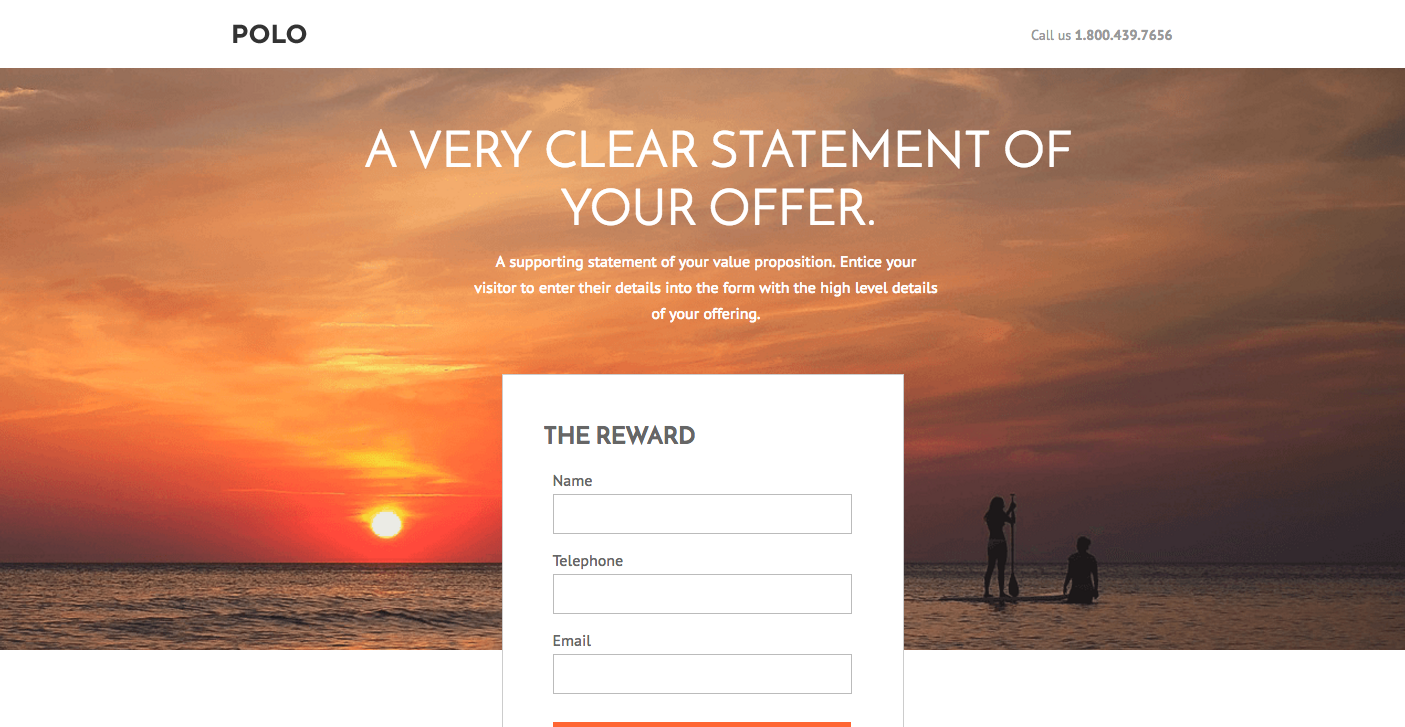A cropped screenshot of a web page, featuring the brand name "POLO" prominently at the top. To the right of the brand name, in small letters, there is a contact number: "Call us 1-800-439-7656." Below this header, there is a large, landscape-oriented image capturing a serene sunset or sunrise over the ocean, with a hazy sky and clouds tinged with glowing orange and yellow hues.

In the middle of this image, there's a text box. To the right of this text box, two people are depicted on a surfboard – one standing and holding a paddle, the other kneeling. Centered within the text box are the words "THE REWARD," followed by input fields labeled "Name," "Telephone," and "Email." Below these input fields is the top edge of a partially visible orange button, likely intended for submitting the form.

Above the text box, in all capital letters, a bold statement declares the core offer, while smaller text underneath provides a supporting statement designed to entice visitors by detailing the value proposition and encouraging them to fill out the form. The overall design combines striking imagery with a clear call to action, aiming to engage visitors and capture their information.